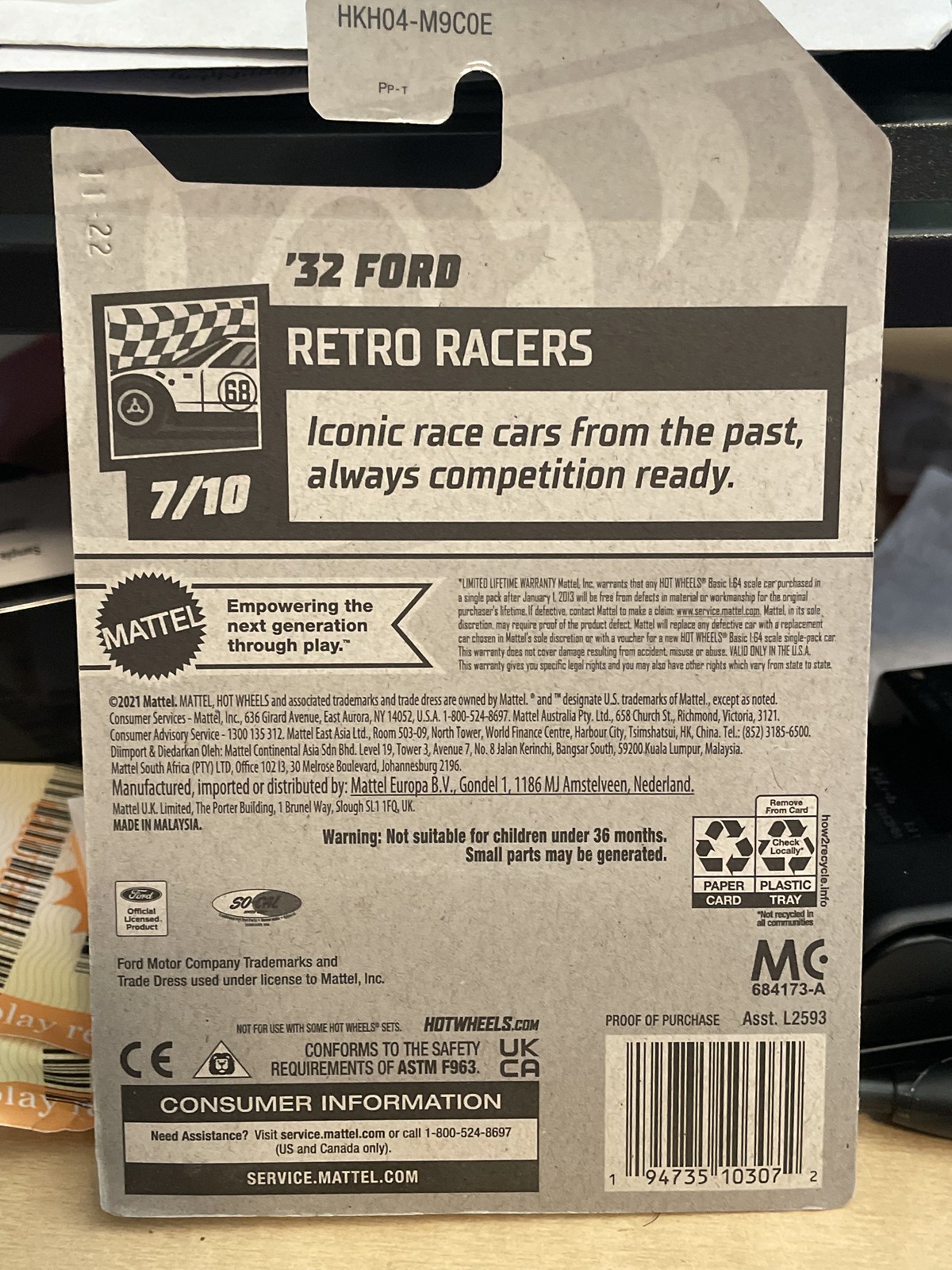The photograph depicts the back of a gray Hot Wheels package for a '32 Ford from the Retro Racers series, numbered 7 out of 10. The top features the title "HKH04-M9COE" and "32 Ford Retro Racers," followed by the tagline "Iconic race cars from the past, always competition ready." Below, there's a graphic of a car with a checkered flag in the background. The Mattel logo is prominently displayed, accompanied by the slogan "empowering the next generation through play." The package also provides detailed information about the manufacturer, Mattel Europa BV based in Amstelveen, Netherlands, and notes that the product is made in Malaysia. It includes warnings that the toy is not suitable for children under 36 months due to small parts. Additionally, the package asserts its status as a Ford official licensed product with Ford trademarks used under license to Mattel Inc. At the bottom right, a barcode and proof of purchase section are visible, featuring the UPC barcode.